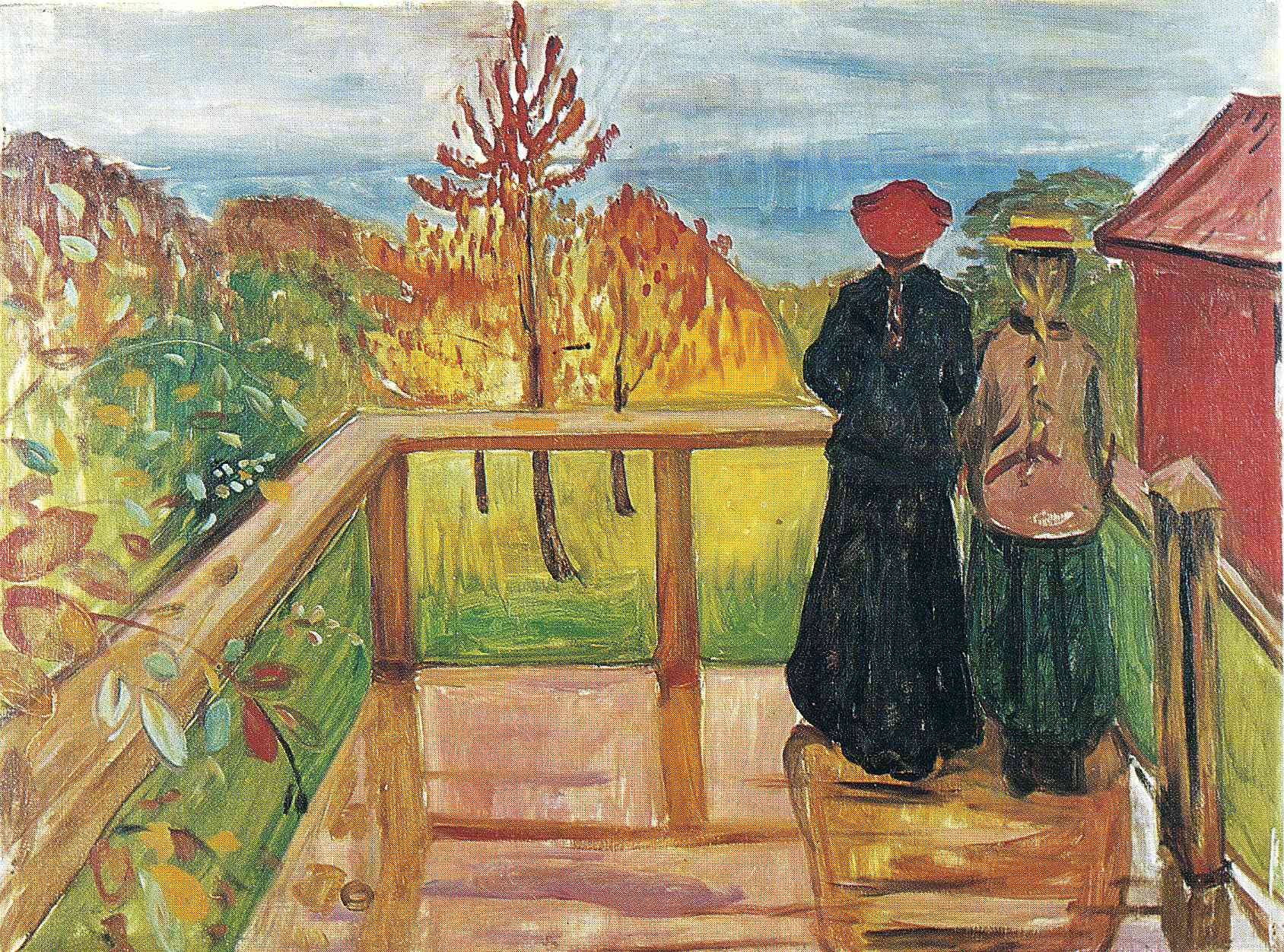The painting, vivid and colorful, captures two women standing on a pinkish wood porch, gazing out at a picturesque landscape. The artwork, done in acrylic, has a stylized, slightly abstract quality. The women, dressed in Victorian-era attire with long dresses reaching their ankles, have their backs turned to us. The taller woman on the left sports a dark green dress, a red hat, and long brown hair tied in a ponytail. Her companion, slightly shorter, wears a black sweater and black dress, paired with a light yellow hat, and has blonde hair, also tied in a ponytail. The porch features wooden railings, adding to the sense of an old-time viewing point or balcony.

In the scenic landscape before them, a red barn with a matching roof stands prominently to the right. The scene is bathed in autumn colors, with vibrant orange and red trees scattered across the green and yellow grasses. The left side of the landscape is particularly lush with additional colorful bushes and greenery. A serene blue sky, dotted with white clouds, stretches overhead, completing the tranquil autumnal setting.